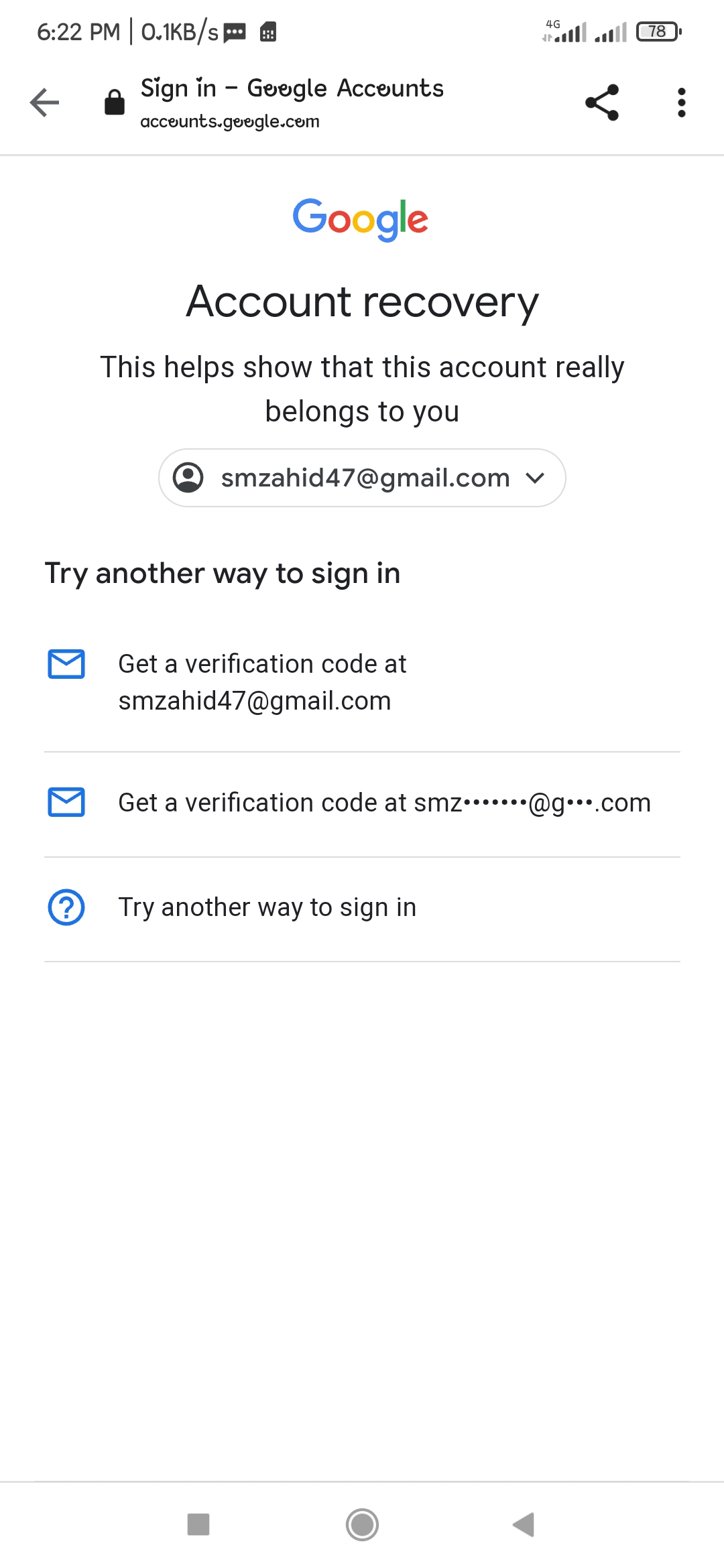This is a detailed screenshot of a smartphone display at 6:22 PM, showcasing various interface elements related to account recovery on Google.

**Top Bar Elements:**
- Time displayed as "6:22 PM."
- A vertical line separator.
- Data transfer rate listed as "0.1 KB/s."
- Three vertical dots indicating a menu option.
- Signal strength displayed as "4G" with full bars.
- Battery icon showing "78%."

**Main Screen Content:**
- A left-facing arrow icon followed by a padlock symbol.
- Large text stating "Sign in - Google Accounts."
- Below, in smaller font: "accounts.google.com."
- On the right side, three vertical dots indicating another menu option.

**Google Account Recovery Section:**
- The Google logo in its characteristic colors: blue, red, yellow, green.
- Text below the logo reads "Account Recovery," with "recovery" starting with a lowercase 'r.'
- Smaller text beneath this says, "This helps show that this account really belongs to you."
- The center of the screen displays the email address: "smzahid47@gmail.com."

**Account Recovery Methods:**
1. Option: "Get a verification code at smzahid47@gmail.com" with a blue envelope icon.
2. Option repeated but partially cut-off: "Get a verification code at smz...at g...com" with another blue envelope icon.
3. A blue circle with a question mark and the text "Try another way to sign in."

**Additional Elements:**
- These options are separated by faint lines.
- Further down is a sizable whitespace.
- At the bottom are nondescript icons: a gray square, a gray circle with another circle around it, and a small gray triangle.

The layout is predominantly center-aligned, ensuring the primary focus remains on the recovery options and guiding the user through the process.